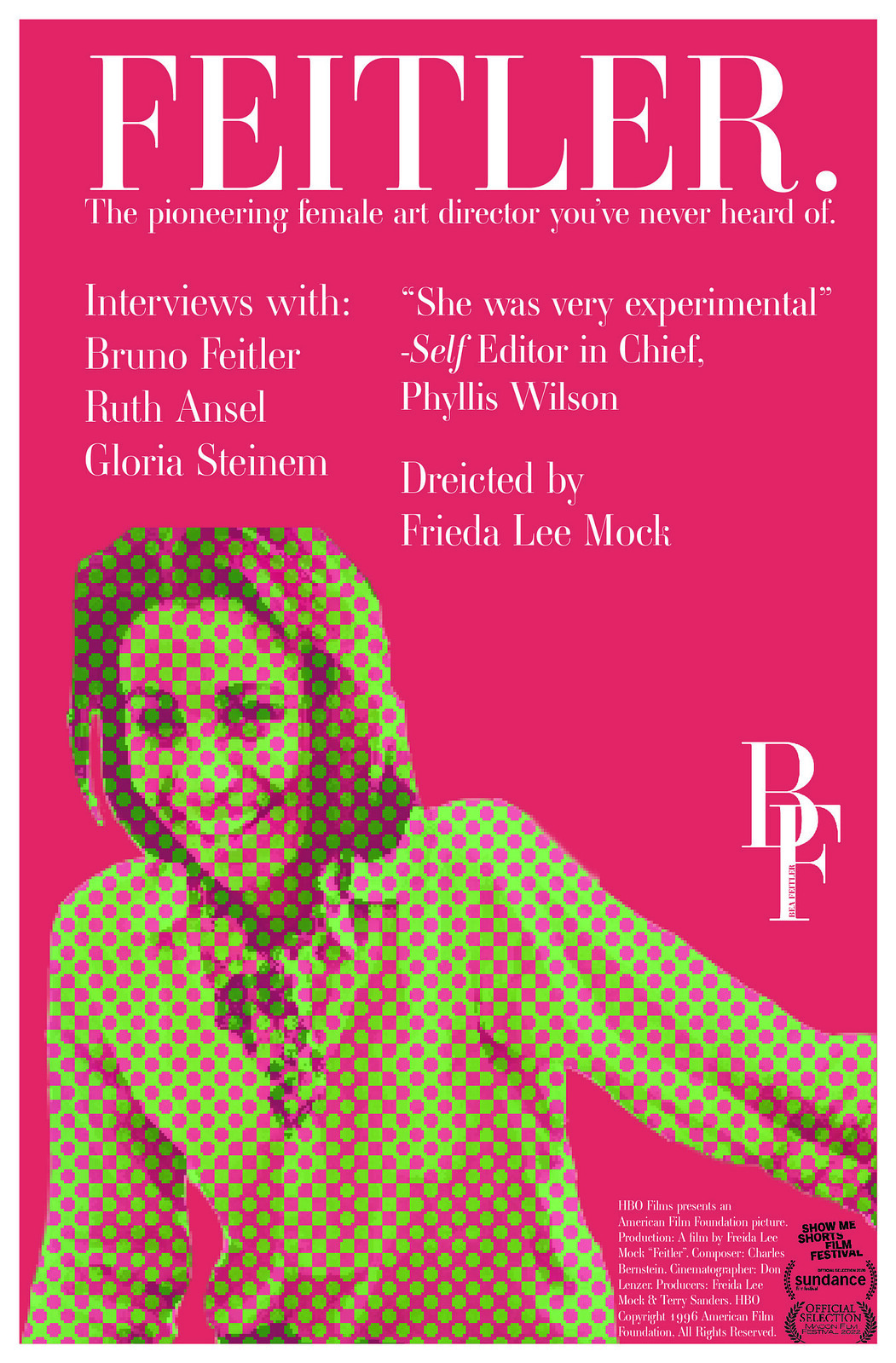The image appears to be a magazine cover with a predominantly red background. The main feature is a blurred photograph of a woman with mid-length or shoulder-length dark brown hair, smiling slightly while leaning forward. She is wearing a white shirt and is distinctively covered in an unusual pattern of green and red dots. 

Above the woman's image, the magazine title "Feitler" is prominently displayed, followed by the subtitle in smaller text: "The pioneering female art director you've never heard of." Beneath this subtitle, the image includes listings for "Interviews with Bruno Feitler, Ruth Ansel, Gloria Steinem," and a quote attributed to the "self-editor-in-chief Phyllis Wilson" noting, "She was very experimental." Additionally, it mentions "Production directed by Frida Lee Mock."

There are also some additional details: a "BF" symbol on the right-hand side of the cover, small white writing at the bottom, and text in the bottom right corner that reads, "Show Me Shorts Film Festival Sundance Official Selection."